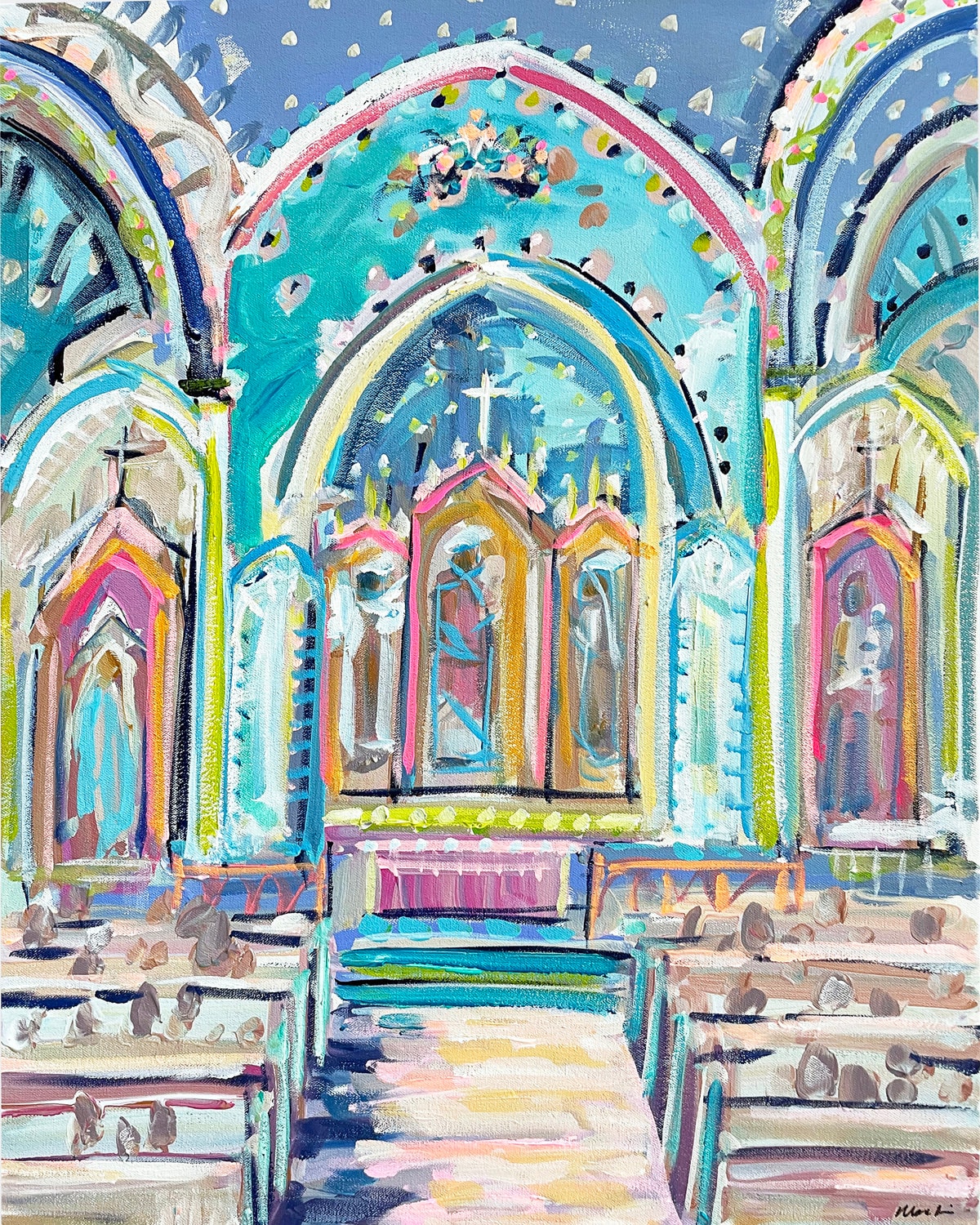This impressionist painting, capturing the interior of a church, is awash with a vibrant palette of blues, pinks, yellows, teals, and oranges, giving it a lively, yet abstract feel. The scene is viewed from the back, looking down the aisle towards the altar. On either side of the aisle are several brown pews, each populated with indistinct figures represented by broad brushstrokes and white highlights, suggesting a congregation of people. Approximately four to five rows of these pews are visible, each holding between three and five heads turned away. Above the pews, the church's walls ascend into ornate arches studded with colorful stained-glass windows, with white crosses crowning the panels that feature depictions of saints and Jesus. The panels and arches combine to create an intricate yet impressionistic representation of a spiritual and sacred space, illuminated by the painting's bright and broad strokes.